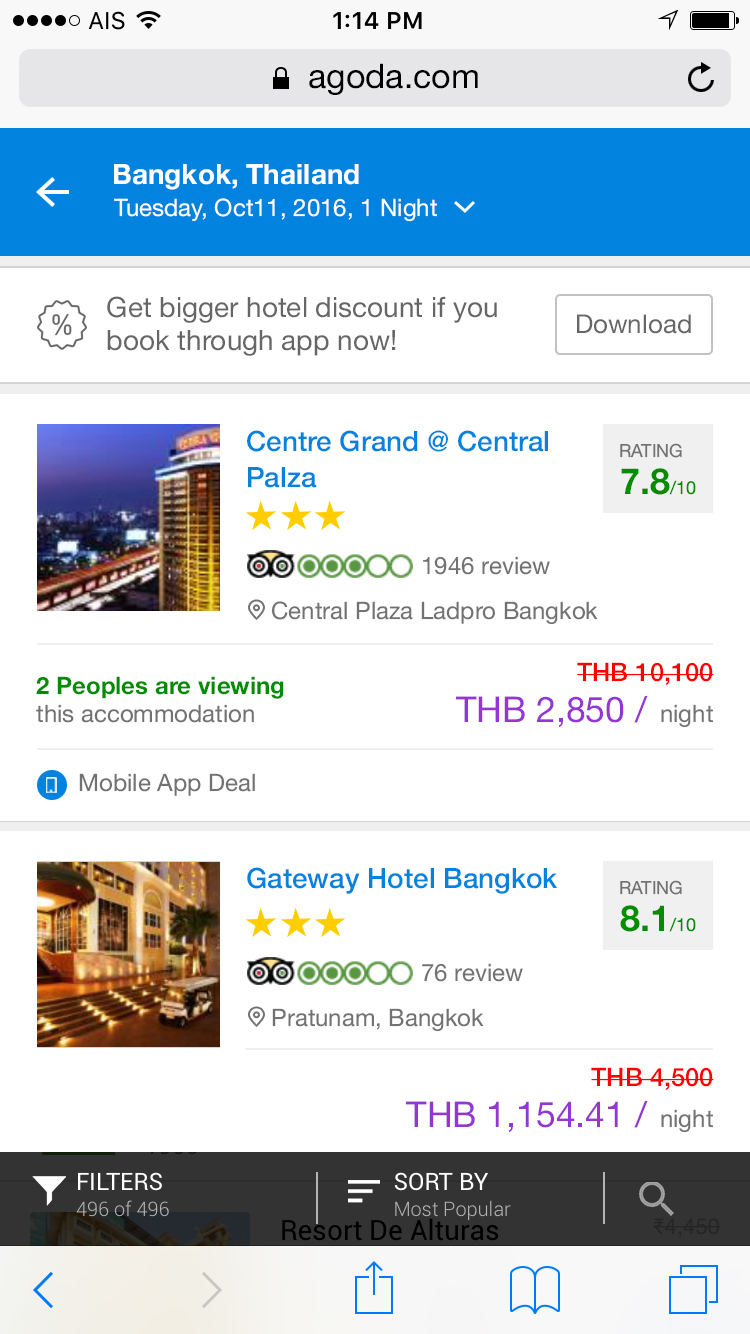A detailed screenshot of a mobile device, possibly a phone or tablet, displaying a webpage is shown. At the top left corner of the screen, there are five dots where four are black and one is white, followed by the logo "AIS" and a Wi-Fi signal indicator. The time in the center reads "1:14 PM." On the top right corner, there is a low battery indicator. The webpage being viewed is agoda.com. 

Beneath this, a prominent blue banner indicates the search criteria: "Bangkok, Thailand, Tuesday, October 11th, 2016, one night," with a white left-pointing arrow on the left edge of the banner. Below this, there's a message in a white background urging users to "Get bigger hotel discount if you book through app now," accompanied by a download button.

Further down, the white background continues with a listing that includes a picture on the left and details on the right: "Central Grand at Central Plaza" is rated 7.8 out of 10 based on 1,968 reviews. The location is "Central Plaza, Lad Prao, Bangkok," and it notes that "Two people are viewing this accommodation."